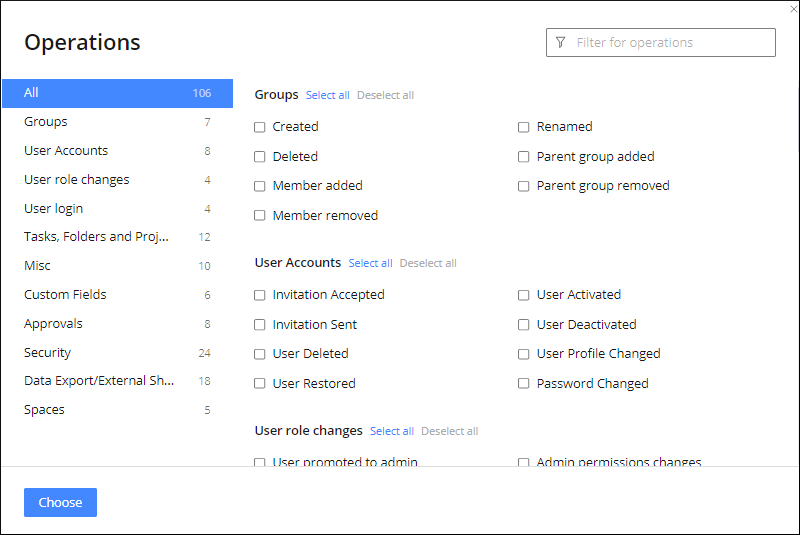This is a detailed screenshot of an administrative panel within an application designed for managing permissions and user groups. The interface features a white background, and the layout is divided into three primary columns.

The first column on the far left is titled "Operations" and lists various operational categories along with their respective counts:
- All (106)
- Group (7)
- User Accounts (8)
- User Role Changes (4)
- User Login (4)
- Tasks, Folders, and Projects (12)
- Miscellaneous (MISC) (10)
- Custom Fields (6)
- Approvals (8)
- Security (24)
- Data Export/External (18)
- Spaces (5)

The middle column displays options to manage groups and user accounts:
- Groups:
  - Select All/Deselect All options
  - Checkboxes for Created, Detailed, Member Added, Member Removed
- User Accounts:
  - Select All (in blue) / Deselect All (in grey)
  - Checkboxes for Invitation Accepted, Invitation Sent, User Deleted, User Restored
- User Role Changes:
  - Select All (in blue) / Deselect All (in grey)
  - Checkbox for User Promoted to Admin

The far-right column provides filters and additional user account-related operations:
- Under "Operations" filter:
  - Checkboxes for Renamed, Parent Group Added, Parent Group Removed
- Under "User Accounts":
  - Checkboxes for User Activated, User Deactivated, User Profile Changed, Password Changed
- Under "User Role Changes":
  - Checkbox for Admin Permission Changes